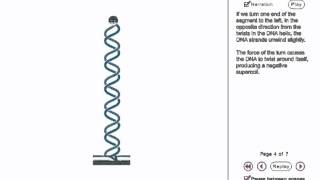This image is a digital screenshot of a page from an ebook or digital document, specifically page 4 of 7. The entire background is solid white. On the left side of the image, there is a diagram consisting of two lines, one gray and one blue, that crisscross and wind upwards. The diagram resembles a screw or spiraling lines. To the right of the diagram, soft black text appears in two somewhat blurry paragraphs, making it difficult to read. Above the paragraphs, there are navigation controls including play, rewind, and fast forward buttons, along with a 'replay' option. Overall, the page layout contains a contrast of black text on a white background with the small addition of green color within the crisscrossing lines or a logo.